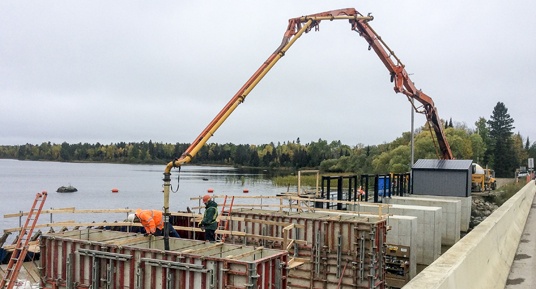The photograph captures a bustling construction site on a dock nestled along the edge of a water body, potentially a lake or ocean, under a cloudy daytime sky. The site is bustling with activity as workers in safety jackets and helmets oversee the project. A large, crane-like machine with yellow and orange tubes towers overhead, seemingly pouring concrete into rectangular molds or containers, likely forming new structures along the shoreline. The foreground shows a prominent concrete wall which acts as a barrier separating the water from a nearby roadway. Additional features include various containers, boxes, railings, staircases, and pillars scattered across the site. In the background, tall trees and hilly terrain covered in greenery provide a scenic contrast to the industrial foreground, while a few boats on the water and the clouded sky complete the vivid, detailed portrayal of ongoing construction near the peaceful, forest-surrounded lake.